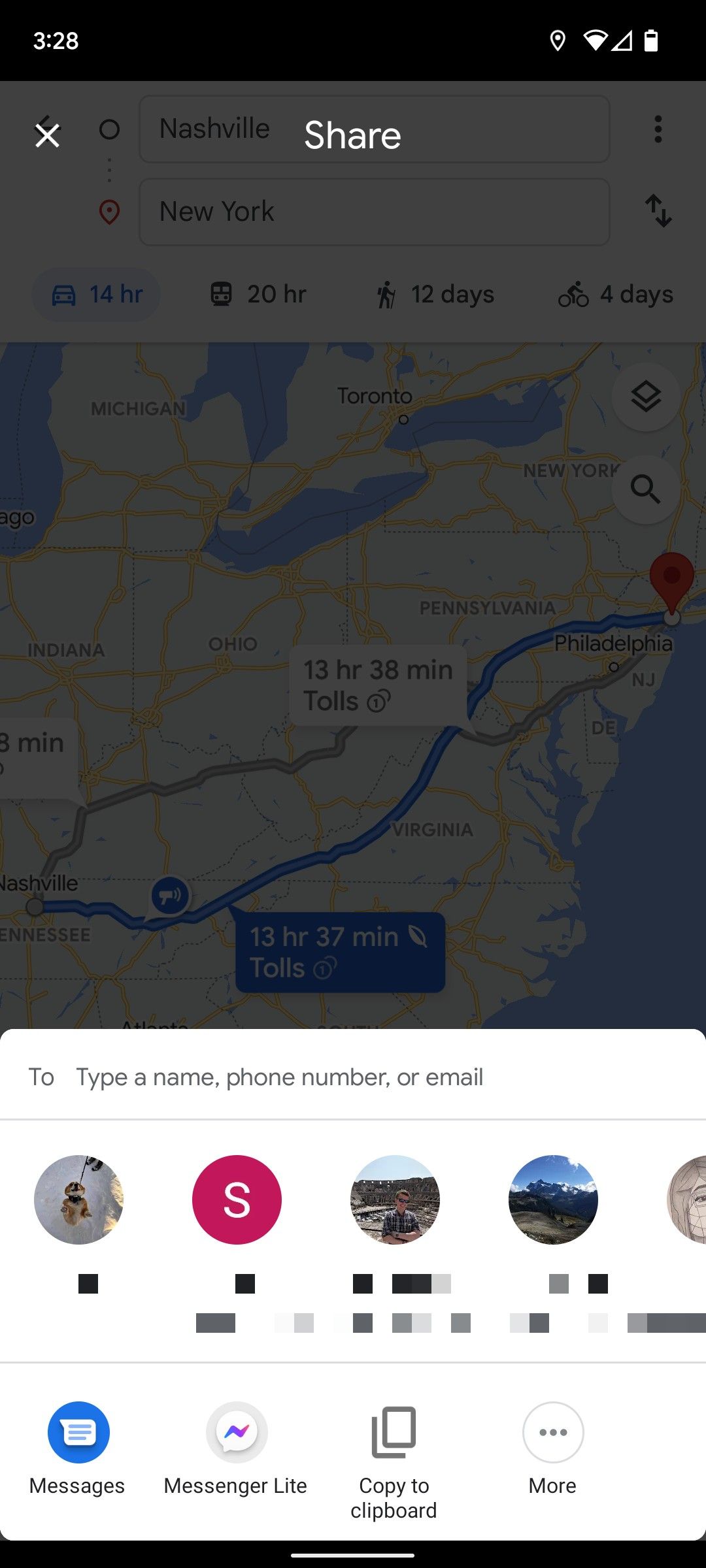In this image, a smartphone displays a Google Maps route charting a journey from Nashville to New York, with an estimated driving time of 13.5 hours. This screen is slightly dimmed as a sharing overlay takes prominence in the foreground. The overlay provides options to share the directions via various apps or contact methods. At the top of the overlay, there is a "Share" header with an option to exit. Below, users can choose from several sharing methods, including messaging apps and copying the link to the clipboard. There's also a search bar to enter a name or number. The visible contacts have their names blurred, but their profile pictures are discernible: one featuring a puppy, another showing a man in sunglasses outdoors, and a third depicting an outdoorsy scene. The "More" button offers additional sharing options.